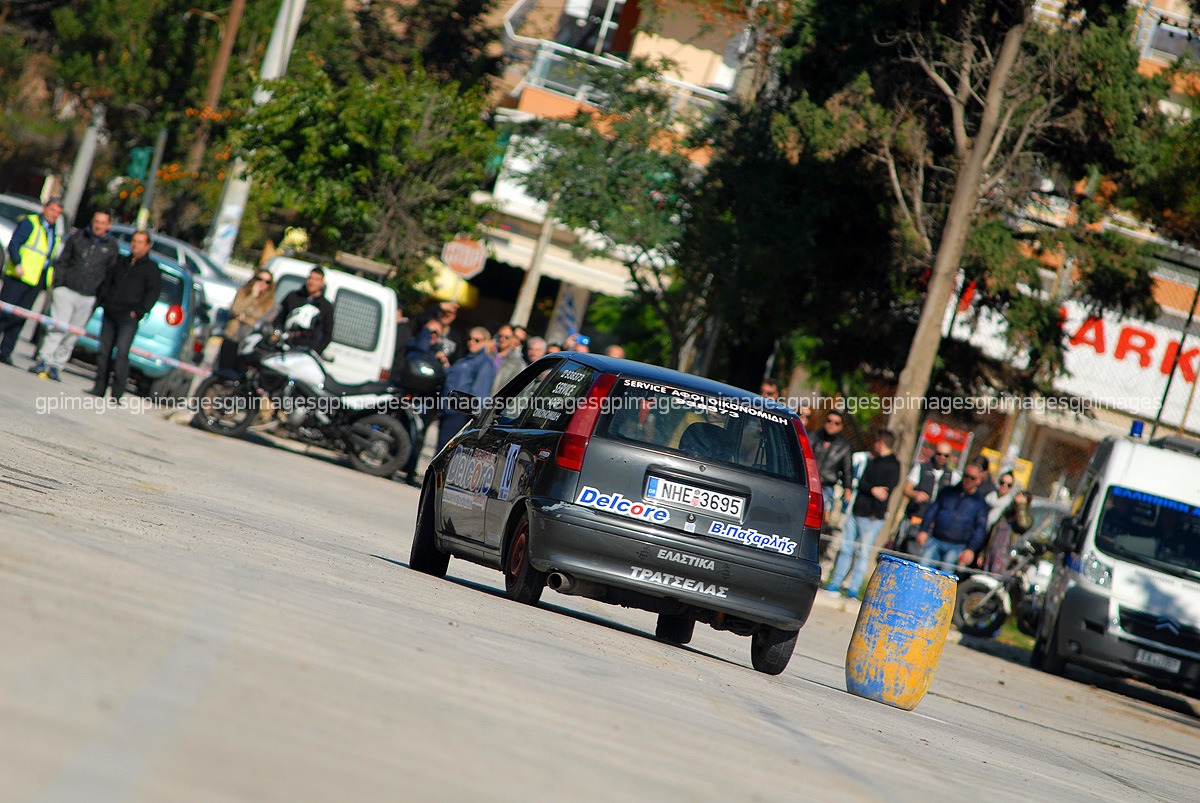In the image, we see a lively town street scene centered around a blue hatchback car marked with the name "Delcor" and a service message written in Greek lettering on the back window. The car, which carries the license plate NHE3695, is captured from its left rear, with only the left taillight visible. Adjacent to the right rear wheel is a weathered barrel, primarily blue with worn edges revealing orange paint beneath. In the mid-ground, there is a crowd of 20 to 30 people gathered behind barricades, seemingly watching the car drive by.

Detailed elements include:
- The crowd includes several individuals in jeans and a man wearing a yellow safety vest.
- A white motorcycle is parked beside the crowd on the right side of the car.
- Storefronts are visible behind the crowd, with one sign reading "ARK" in orange letters against a white background.
- To the right of the barrel, a truck is parked, and a tree stands in front of a building.
- On the left side, another white motorcycle is parked. There are two people standing behind it, near a van, with three more individuals nearby, one of whom is wearing a green safety vest.

The setting appears to be a city street that has been closed off for an event, possibly a car race, as indicated by the barricades and the assembled spectators. The background features an array of buildings, trees, and additional parked vehicles, contributing to the bustling urban ambiance.